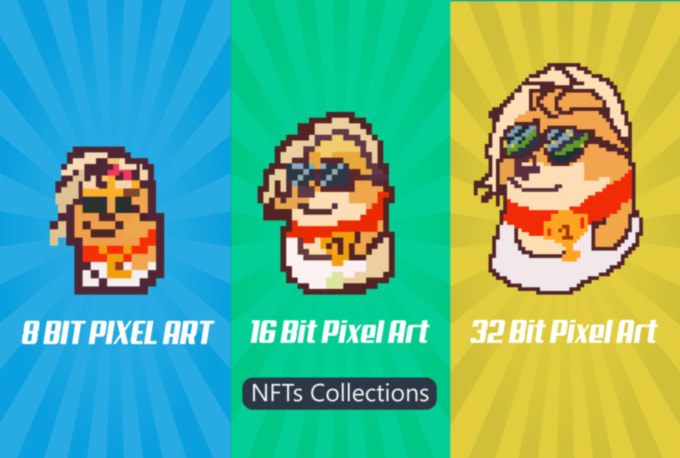This digitally created image showcases a series of three NFTs collections, each with a pixelated depiction of a brown, anthropomorphized animal, possibly a bear, dog, or hamster. The image is divided into three sections, progressing from left to right, and increasing in visual quality:

- **Left Section:** The background is blue with the label "8-bit pixel art." It features a very pixelated image of the brown animal, which appears small compared to the others.
- **Middle Section:** The background is green with the label "16-bit pixel art." The same brown animal is depicted with a slightly higher resolution and is wearing sunglasses.
- **Right Section:** The background is yellow with the label "32-bit pixel art." This section presents the animal in the highest resolution, wearing sunglasses and a red necklace that has a number one trophy hanging from it.

The text "NFTs Collections" is noticeable, indicating that these images are part of NFT series. The animals increase in size and pixel clarity from left to right, showcasing the evolution of pixel art through 8-bit, 16-bit, and 32-bit graphical styles. The color palette includes shades of red, brown, tan, beige, green, light blue, gold, yellow, and black. Each detail, from the sunglasses to the trophy, highlights the distinct features and settings of each artwork within the collection.